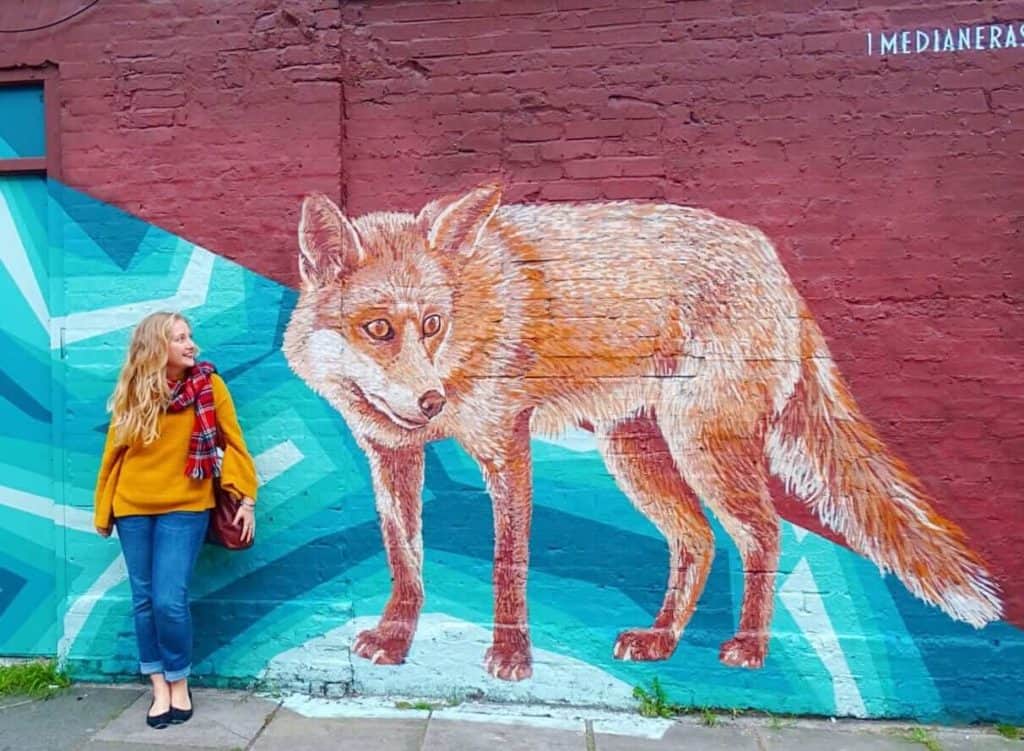In the image, a young Caucasian woman with long blonde hair stands on a gray sidewalk, where patches of grass grow in the cracks, in front of an old, slightly worn red brick building. The building features a large, vibrant mural. To the right of the woman, the mural showcases a massive fox, painted in shades of orange, brown, and white, with strikingly large eyes gazing to the right away from the viewer. The fox stands on a boldly colored geometric design comprising white, teal, blue, and dark blue elements, topped with zigzagging patterns that extend from the building down to the sidewalk. The woman, who appears to be captivated by the mural, wears a yellow sweater, a red and black plaid scarf, blue jeans, and black shoes. She also carries a brown pocketbook over her shoulder. A door painted as part of the mural is located to her left, blending into the overall artwork.